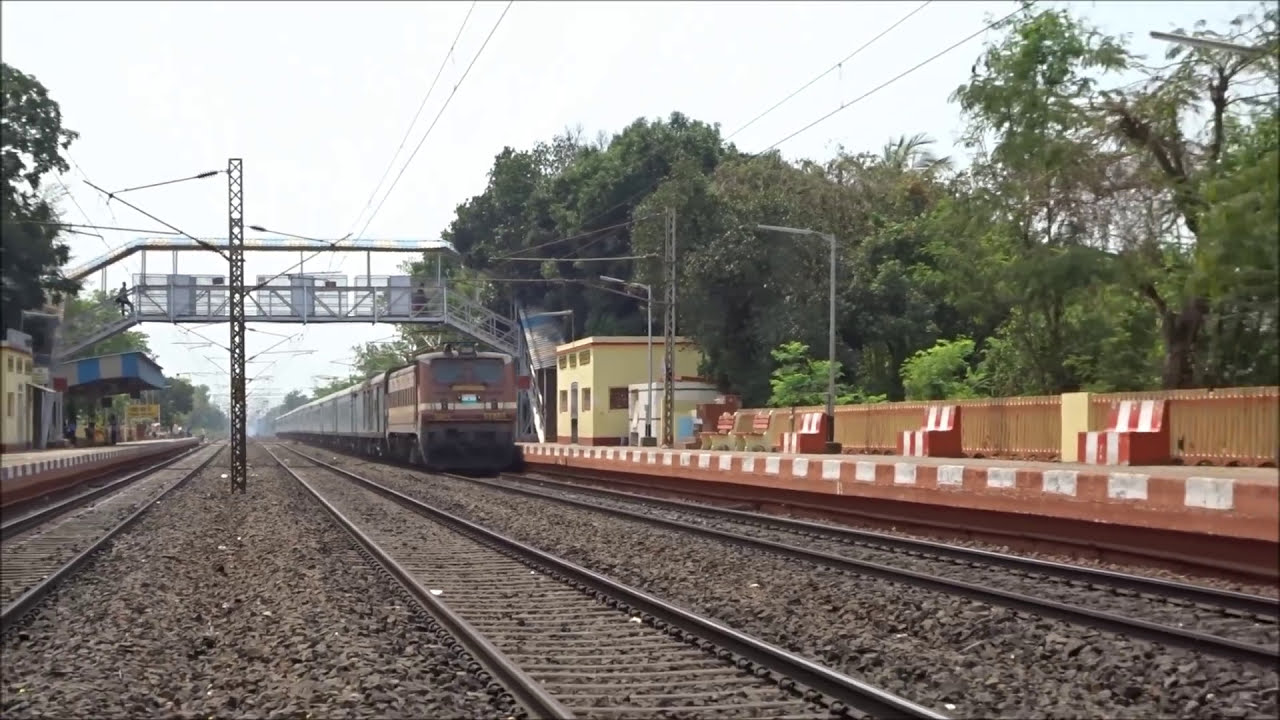The photograph captures an outdoor scene at a bustling train station under a predominantly gray sky. Dominating the image is a train with a brown front, making its way along the multiple train tracks that crisscross the scene, their foundation composed of scattered rocks and pebbles. Around the midsection of the photo, a metal catwalk spans from one side to the other, with a solitary pedestrian crossing. The station is bordered by numerous trees, rich with green leaves, and flanked by power lines.

On the far right, a platform is visible, furnished with brown and white striped, and possibly somewhat brick-red, benches for waiting passengers. Among them, a few people wait for the arriving train. Adjacent to this, a yellow building stands out against the verdant backdrop. There is also a fence visible in the distance. The overall atmosphere suggests an everyday moment at a lively train station, with passengers anticipating the train's arrival amidst a picturesque, tree-lined setting.